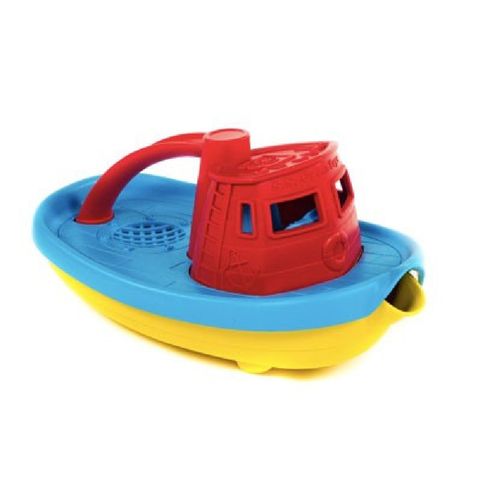The image depicts a colorful plastic toy boat set against a white background, likely digitally enhanced. The boat is designed for children's play, possibly to make bath time more enjoyable. The top section of the boat is blue, while the bottom is yellow. The toy features an orange front section, resembling a ship's head, which includes two large front-facing windows and a small side window on each side. A red cockpit is situated on top, containing a ladder on the left side and two large front windows providing a clear view ahead. From the back of the cockpit, a slide extends down to the yellow base of the boat. The boat also includes functional elements, such as a mesh floor at the rear to allow water drainage and a spout at the front for pouring water, making it versatile and interactive for children.